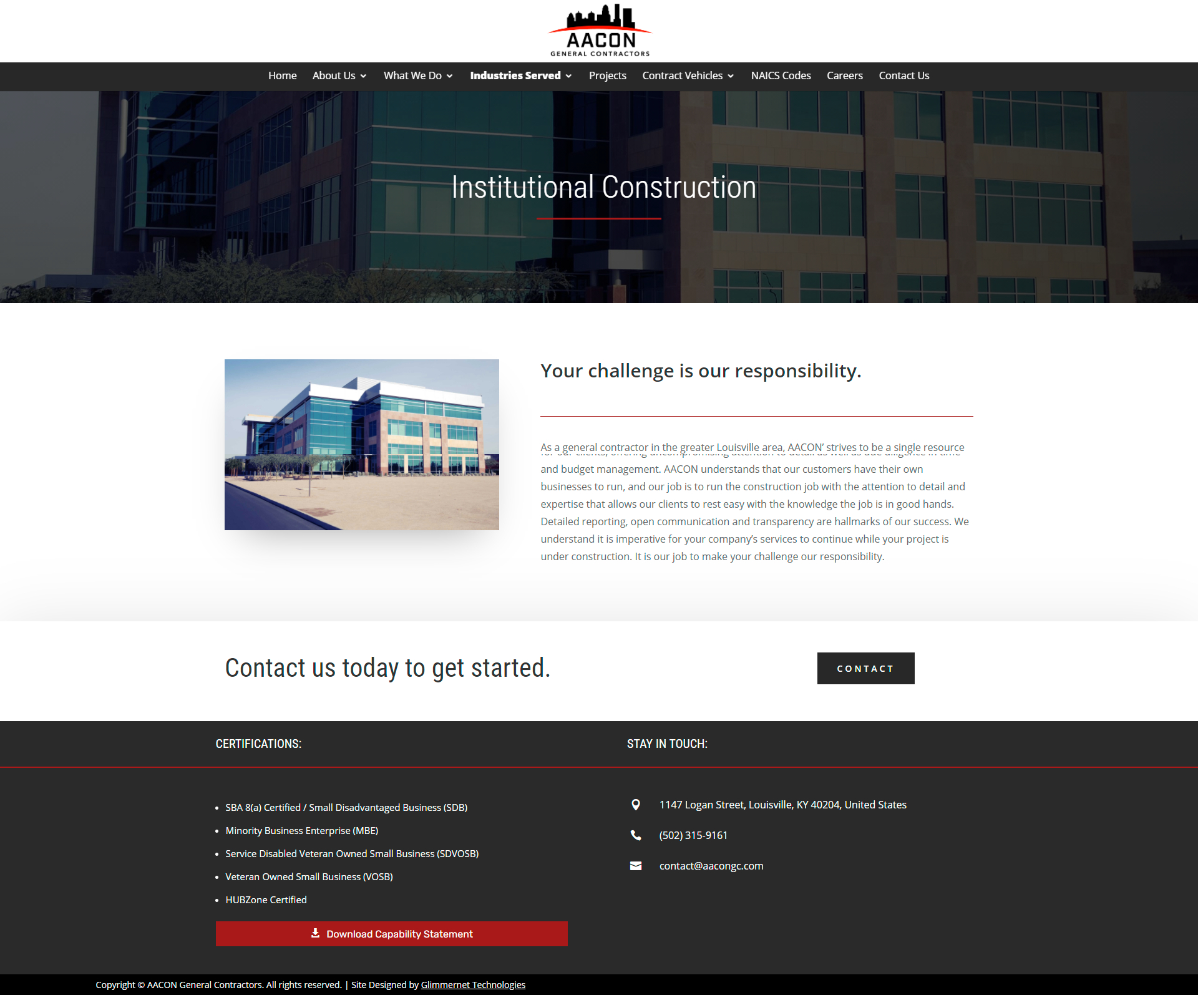This rectangular screenshot features the website layout of AECON General Contractors. At the top of the image is a solid white header displaying AECON's logo, which depicts a city skyline. Below the white header, there is a deep gray banner running horizontally across the top of the page. Within this banner, the words "Institutional Construction" are prominently displayed. The navigation menu includes options such as "Home," "About Us," "What We Can Do," with "Industries Served" being highlighted.

On the left side of the layout, there is a small photograph depicting a large office building during daytime. The building is primarily made up of glass windows and doors. Adjacent to this image, it states: "Your Challenge is Our Responsibility. As a general contractor in the Greater Louisville area, AECON strives to be a single resource and budget management. AECON understands that our customers have their own businesses to run and our job is to run the construction job with the attention to detail and expertise that allows our clients to rest easy with the knowledge the job is in good hands."

Below the photograph and the accompanying text, there is a call-to-action: "Contact us today to get started." Further down, the sections "Certifications" and "Stay in Touch" are visible, encouraging potential clients to learn more about AECON's credentials and to engage with the company.